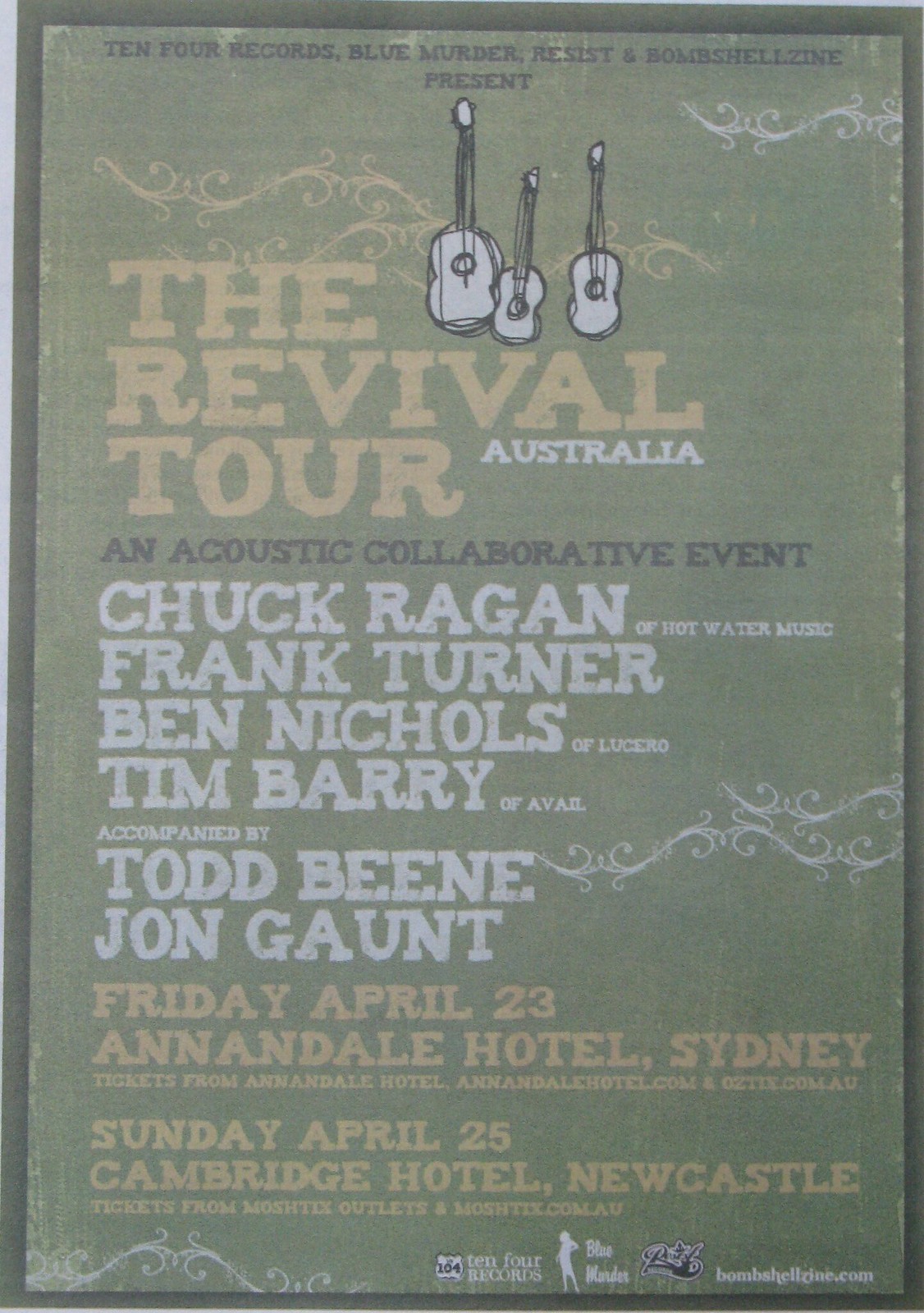The poster has a vintage aesthetic reminiscent of designs from the 1930s or 1940s, featuring a dark green border and a light green background. At the top, it announces in black text "10-4 Records, Blue Murder, Resist, and Bombshellzine Presents." Below this, three illustrated guitars are arranged in a row, emphasizing the musical theme. Prominently in yellow bold letters, it says "The Revival Tour," with "Australia" in white text underneath. Following this, in black text, it states "An Acoustic Collaboration Event." The poster lists the performers in white text: "Chuck Regan of Hot Water Music, Frank Turner, Ben Nichols of Lucero, Tim Berry of Avail, accompanied by Todd Bean and John Gaunt." At the bottom, in an orange-beige hue, it details the event dates and venues: "Friday, April 23rd, Annandale Hotel, Sydney. Tickets from Annandale Hotel, annandalehotel.com," and "Sunday, April 25th, Cambridge Hotel, Newcastle. Tickets from Moshtix Outlets and moshtix.com.au." Although it gives the impression of being an old-school design, the inclusion of website URLs confirms that it is a modern poster intentionally styled to look vintage.